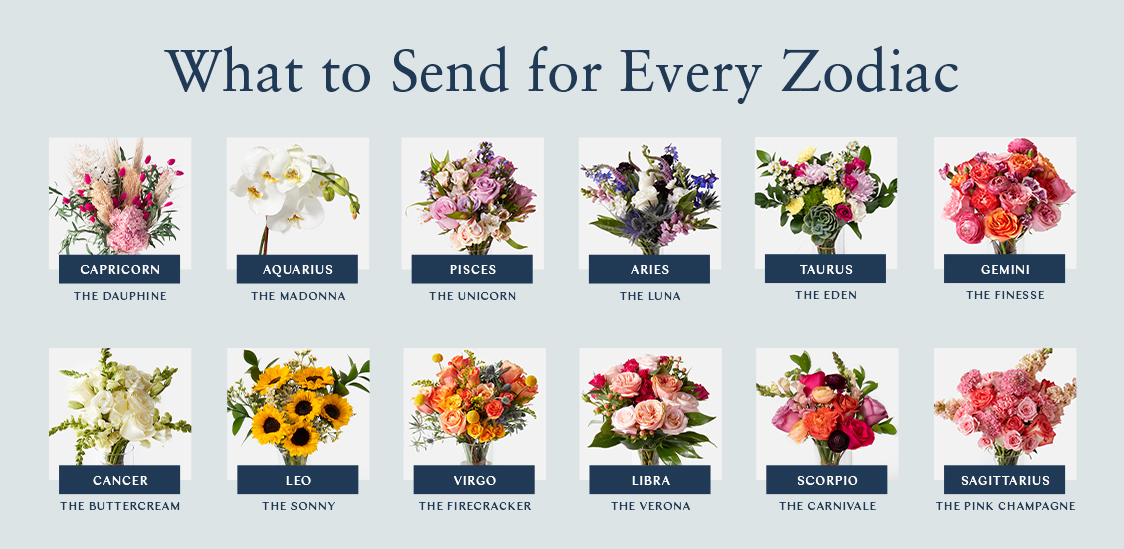This digitally synthesized image features a light gray background and is designed as a poster titled "What to Send for Every Zodiac," written in large navy text centered at the top. Below the title are two rows of six evenly spaced photos of flowers, each with a white background and a navy bar underneath displaying the corresponding zodiac sign in white text. Beneath each flower's image, the name of the flower is listed. 

For the top row, from left to right:
1. **Capricorn** - A bouquet of white, pink, and brown flowers labeled "The Dauphine."
2. **Aquarius** - A white orchid labeled "The Madonna."
3. **Pisces** - A bouquet of purple and white flowers labeled "The Unicorn."
4. **Aries** - A bouquet of white, purple, and blue flowers labeled "The Luna."
5. **Taurus** - A bouquet of green, yellow, pink, and white flowers labeled "The Eden."
6. **Gemini** - A bouquet of orange, red, pink, and purple flowers labeled "The Finesse."

For the bottom row, from left to right:
1. **Cancer** - A bouquet of white flowers labeled "The Buttercream."
2. **Leo** - A bouquet of sunflowers labeled "The Sunny."
3. **Virgo** - A bouquet of yellow, orange, and red flowers labeled "The Firecracker."
4. **Libra** - A bouquet of pink, white, and light pink flowers labeled "The Verona."
5. **Scorpio** - A bouquet that has dark purple, light pink, orange, and yellow flowers labeled "The Carnival."
6. **Sagittarius** - A bouquet of red, pink, and white flowers labeled "The Pink Champagne."